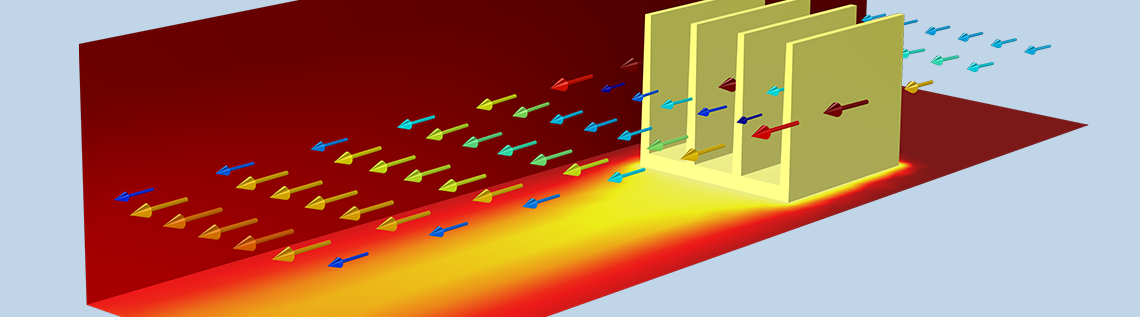The image is a detailed industrial-style vector illustration reminiscent of classic Macromedia Freehand or Adobe Illustrator techniques. Set against a light blue background, a geometric, light yellow object sits prominently in the center, resembling a tabletop organizer or napkin holder with three compartments made up of four standing walls. The object, which is open on the top and has a golden glow emanating from it, appears to be placed on an indeterminate surface within the blue background. About halfway up the illustration, an array of colored arrows—yellow, green, blue, and red—emerges, traveling from the back left to the front right of the frame. These arrows, barrel-shaped and varied in size, seem to convey a sense of motion or airflow around and through the compartments of the organizer. The image, possibly mimicking airflow or data transfer within a system, features an orange and yellow pattern near the bottom that might signify movement or heat dissipation, suggesting a digital or computational function.